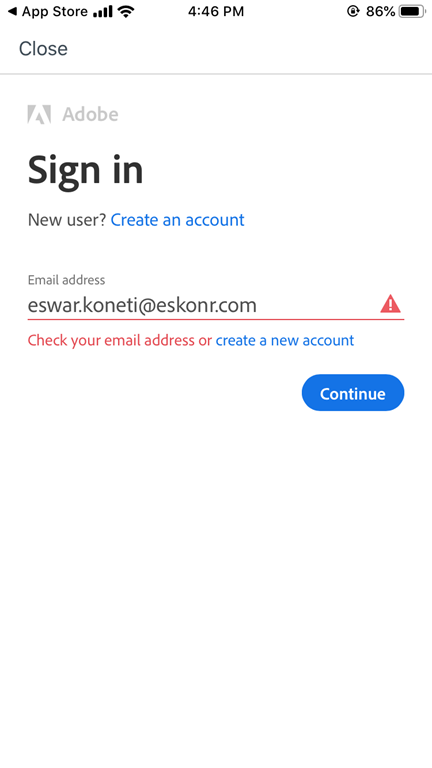The image showcases a smartphone screen displaying the App Store. At the top, the status bar indicates the time as 4:46 p.m., Wi-Fi signal strength, and an 86% battery charge. Below the status bar, a gray line separates the top from the rest of the screen.

Beneath this line, the Adobe logo appears prominently. Following the logo, bold text reads "Sign In." Below this, a question is posed in blue text: "New user? Create an account."

The email address entered is "war.conetti@escrownar.com," which is underlined in red, signaling an error. A red warning message states, "Check your email address or create a new account."

The options to "Check your email address" in red and "Create a new account" in blue are provided for further action. All of this information is displayed against a clean, white background, with no other elements present.

The overall presentation is clear and concise, aiding in user navigation and error correction.